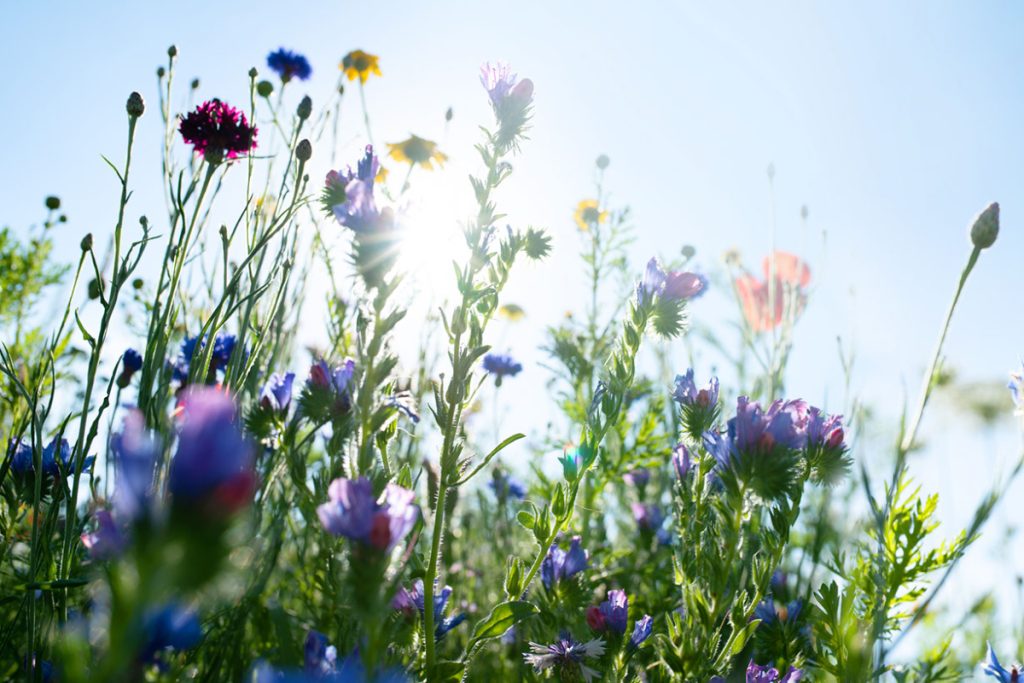This vibrant image captures a breathtaking field of wildflowers from a unique, ground-level perspective, looking upwards through the dense stems toward the sky. The scene is bathed in the warm glow of sunlight peeking through the lush green foliage, casting gentle sun rays on the slender stems. The bright blue sky frames the background, deepening at the edges while a nearly white, sunlit area radiates in the center, highlighting the rich variety of blooms.

A colorful tapestry of flowers punctuates the scene: delicate yellow-petaled flowers mingle with thin-petaled purple ones, vibrant blue blossoms, and striking red flowers, creating a kaleidoscope of hues. The heights and sizes of the wildflowers vary, with some tiny, almost miniature blooms juxtaposed against larger, more prominent flowers, particularly noticeable in the bottom right corner where a few larger red flowers stand out. The overall impression is one of abundant springtime splendor, amplified by the expansive field suggested in the distance, capturing the essence of a day bursting with life and color.